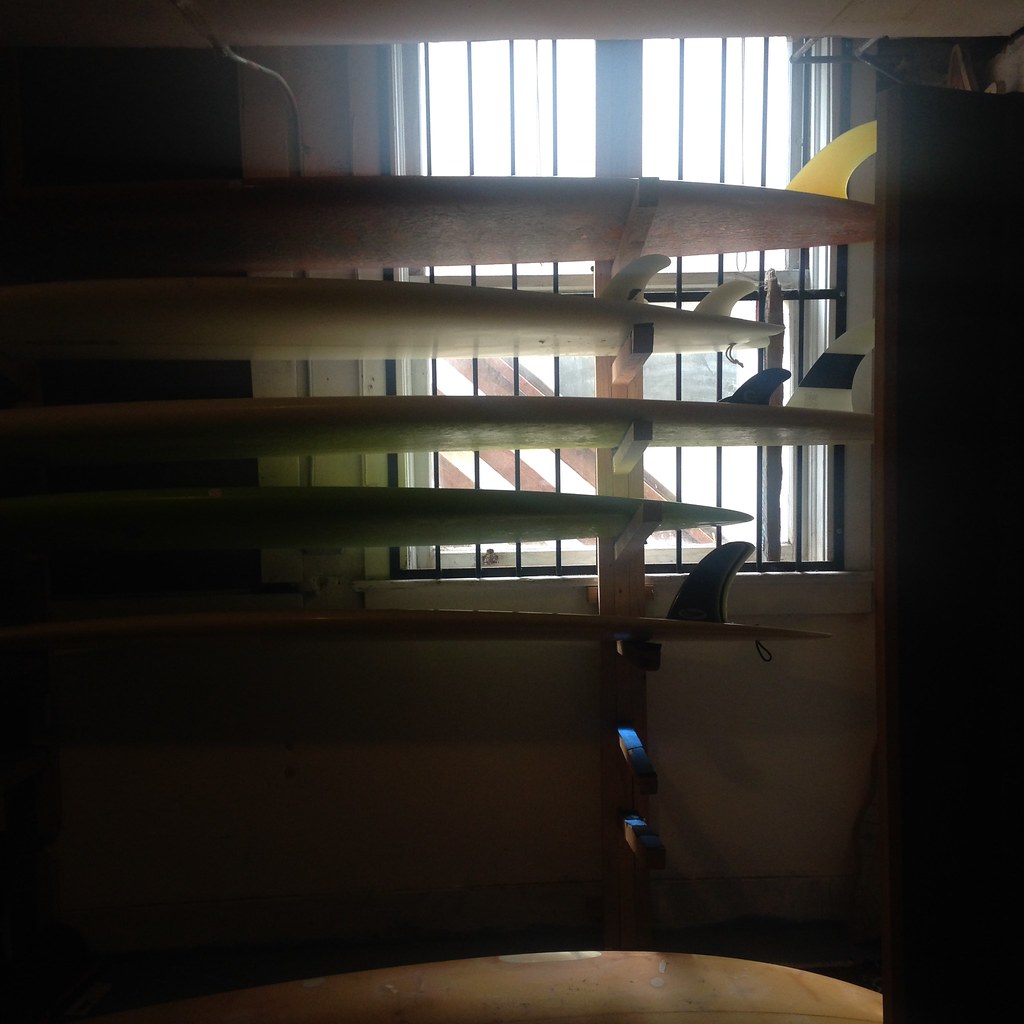This detailed color photograph, taken indoors, captures a shadowy room with a window in the background. The window, featuring black metal grating and partially open slotted lines, allows streams of light to filter in, casting subtle reflections. The wall surrounding the window has a tan hue. In front of the window stands a vertical wooden post with multiple pegs extending horizontally. These pegs hold five surfboards arranged in a stacked formation. The surfboards vary in length, with the sequence from top to bottom being: long, short, long, short, and short again. Notably, the top three and the bottom surfboards have visible fins, while the fourth does not. Beneath these surfboards, the lower pegs are empty. Additionally, a white surfboard is seen resting on the floor, leaning against the wall. The overall ambiance of the photograph is dark and moody, with the window acting as the primary light source.